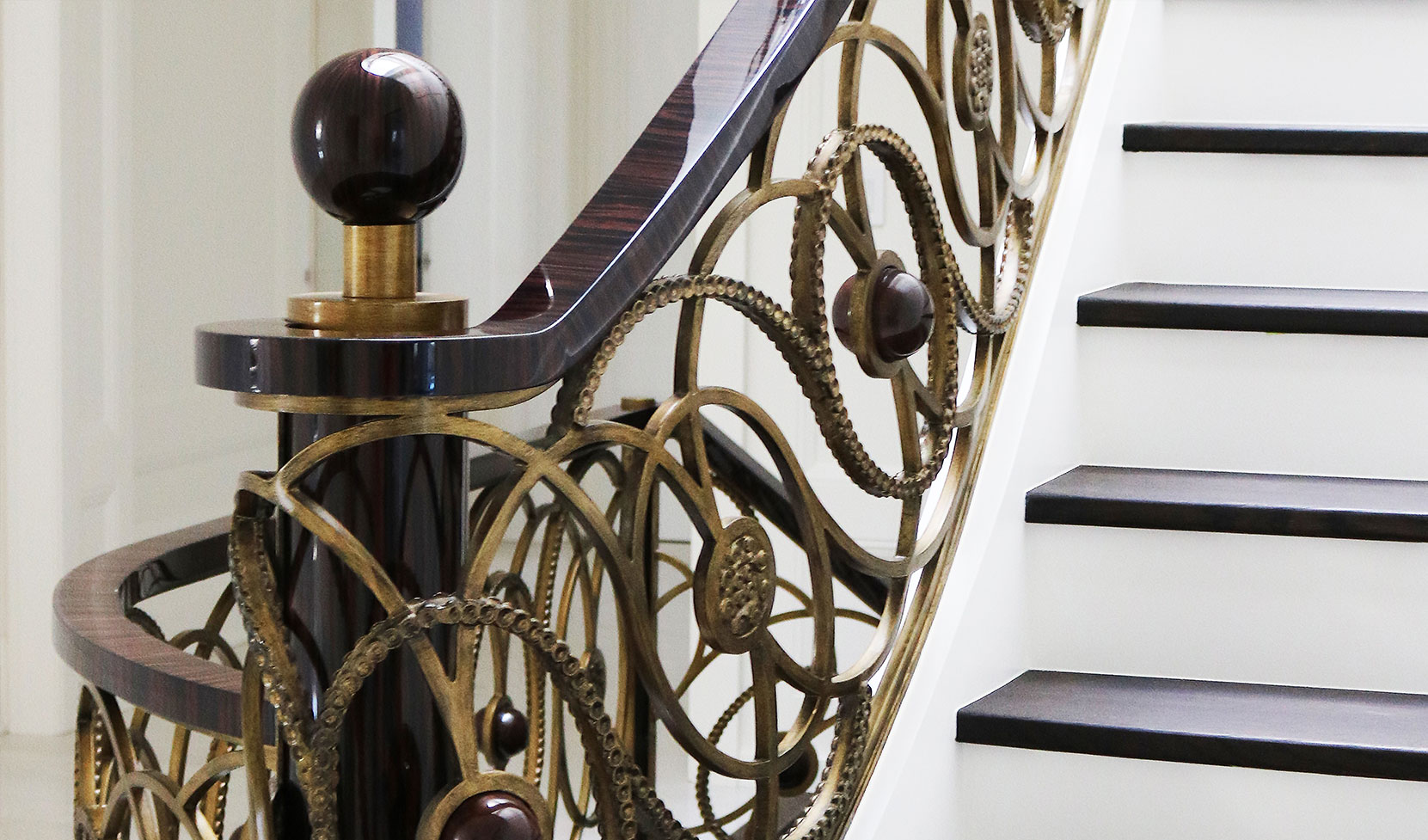This image depicts an elegant staircase of a high-end building, possibly a home or an office. The steps feature a striking design with a dark, likely black, wooden top surface contrasted by pristine white sides. The banister running alongside the staircase is an intricate piece, predominantly black and highly polished, reflecting the surrounding white walls. Adding to its sophistication, the banister incorporates both black and golden intertwined coils, forming a woven pattern that adds a touch of luxury. At the base of the staircase, where the banister curves, sits a large decorative brown orb. Additional smaller brown orbs are encased within the ornate gold and black circular designs along the banister. The overall aesthetic is one of refined elegance, marked by the shiny surfaces and thoughtful contrast of colors.